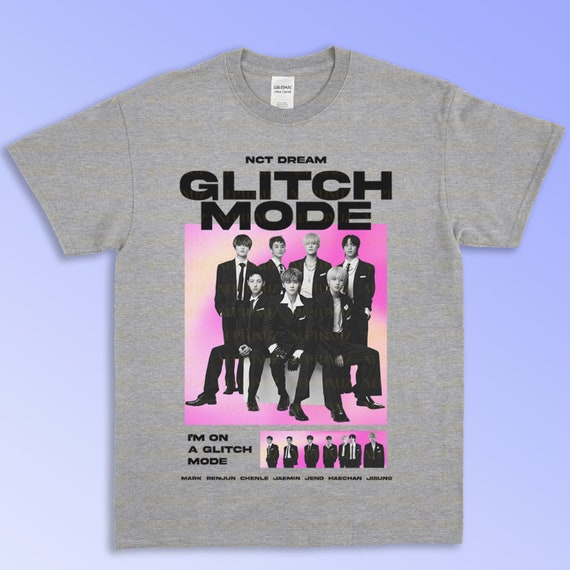The image features a light gray Gildan t-shirt set against a gradient background that transitions from white in the bottom left corner to blue in the top right corner. Prominently displayed on the shirt is an image of the K-pop band NCT Dream. The band members, seven in total, are depicted with four standing in the back and three sitting in front, all dressed in coordinated black suits with a white and pink backdrop behind them. At the top of the shirt, the words "NCT Dream" are printed in small text, followed below by the bold, all-caps title "GLITCH MODE." Underneath the band's image, the phrase "I’m on GLITCH MODE" is also printed in all caps. Additionally, there is another smaller version of the image of the band at the bottom of the shirt, accompanied by the names of the members, though the text is too small to read clearly.